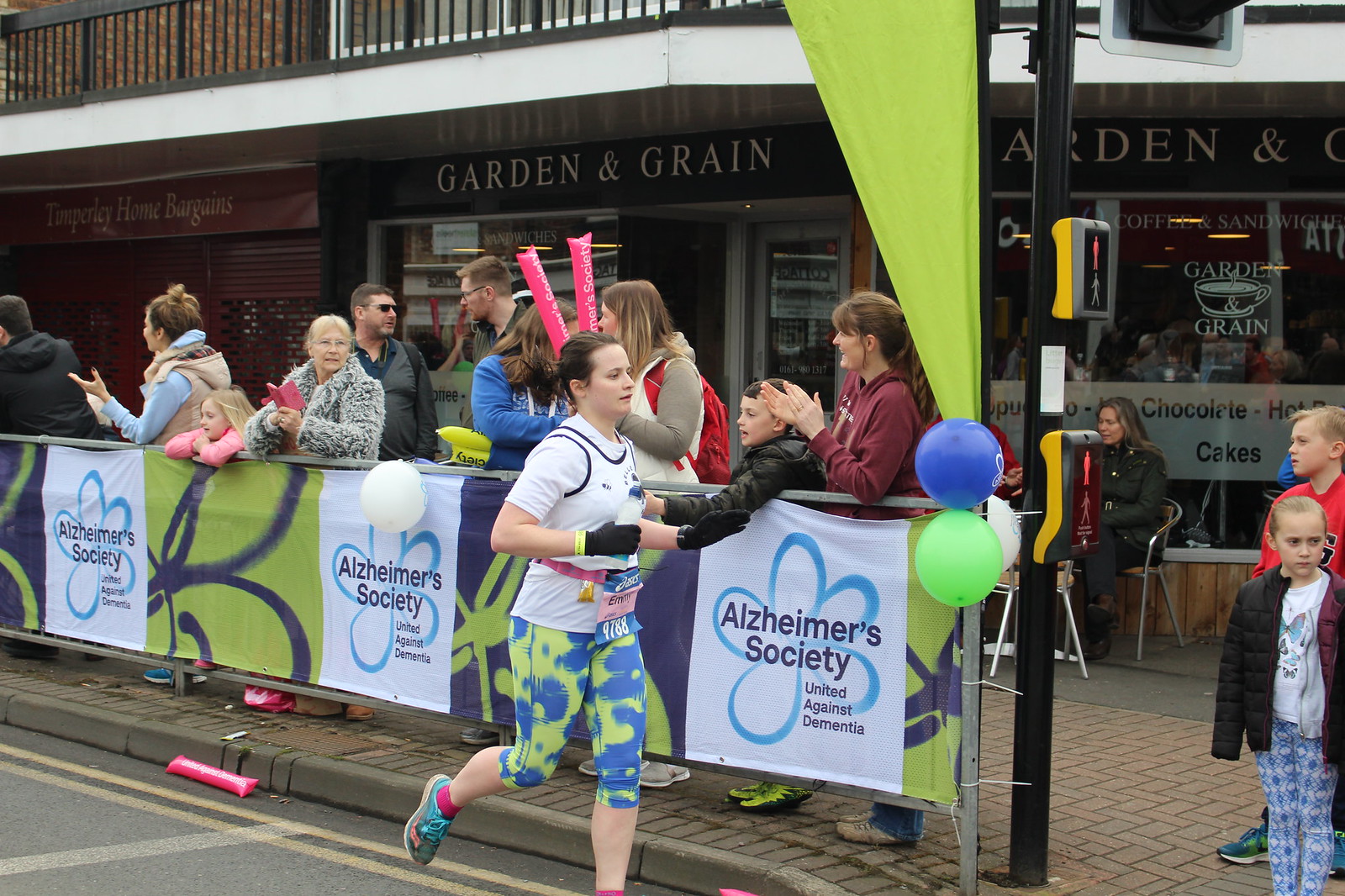In this detailed daytime photograph of a charity road race sponsored by the Alzheimer's Society, a young female runner is captured mid-stride along an asphalt street marked by double yellow lines and a white rectangular line. She wears tie-dye blue and green leggings that end at her knees, brightly colored running shoes, pink socks, black gloves, a white short-sleeved t-shirt layered under a jersey with black piping, and her brown hair is styled in a ponytail.

The foreground features a barricade with a banner displaying the Alzheimer’s Society United Against Dementia slogan, separating the spectators from the runners. Enthusiastic onlookers, including men, women, and children dressed in hoodies and jackets suggestive of cold weather, cheer and reach out towards the runner, possibly for high-fives. 

Behind the crowd, a row of storefronts includes the eatery "Garden and Grain," its name prominently displayed in gold lettering. A woman is seated by the window of this shop. Another store, "Home Bargain," features red signage. Above these establishments, a second-story balcony with a black railing spans the scene.

In the street, near the runner, are two balloons—one green, one blue—tied to a post, matching the color scheme of her attire. A long pink object, possibly an inflated noisemaker, lies on the road, contributing to the vibrant race atmosphere.